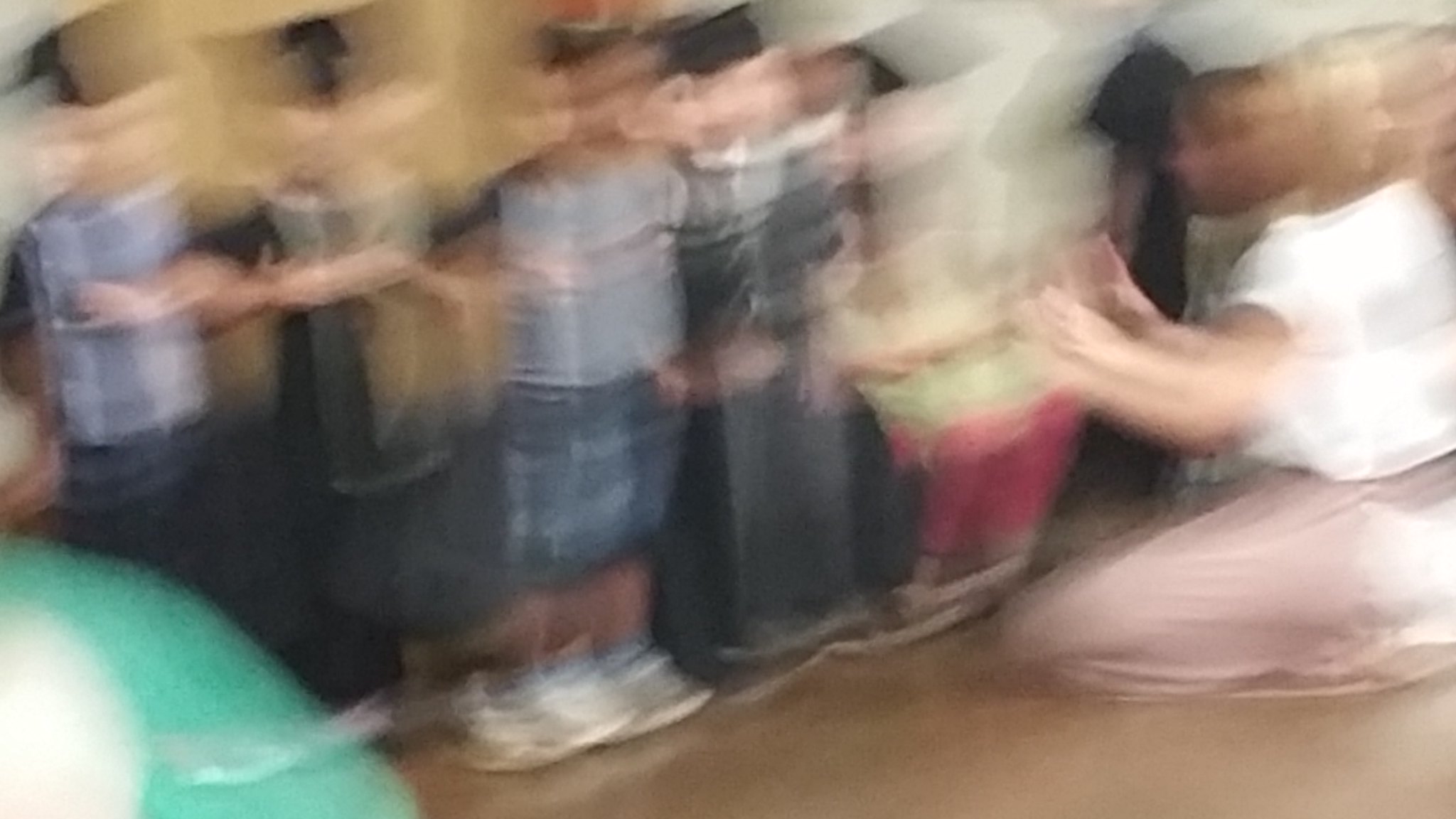In this highly blurred image, a group of children appears to be lined up on the left side. Despite the double exposure effect making details indistinct, one can make out various colors in the children's clothing, including red, yellow, black, blue, and white. They exhibit different skin tones, but the blur obscures finer details. Facing the children, a woman is kneeling on the floor to the right. She has light skin, blonde hair, and is dressed in a short-sleeved white blouse and a light-colored skirt that seems to be beige or very light brown. The floor beneath them is a brown hue. Additionally, a faint, ghost-like adult face is barely visible in the top right corner of the image, although it is heavily blurred.